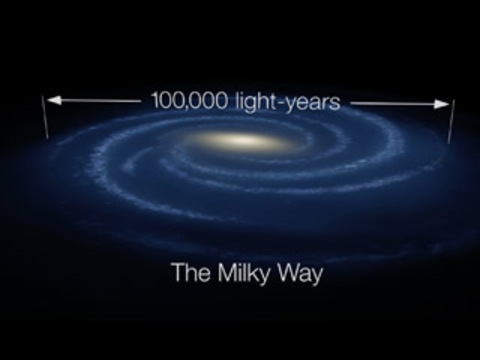The image is a detailed diagram of the Milky Way. It features a predominantly black background, emphasizing the vastness of space. Central to the image is a depiction of the Milky Way galaxy, illustrated with swirling clouds in hues of blue, gray, and black. At the core of the galaxy, there's a bright, glowing light, possibly representing the central bulge or the galactic core, and it emits a yellowish-white radiance. Above this central galactic image, two vertical white lines stand approximately two inches tall, flanking each side of a pair of arrows that span horizontally from one line to the other. Between these arrows, the text "100,000 light-years" is prominently displayed, indicating the scale of the Milky Way's diameter. Beneath the swirling galactic image, the text "Milky Way" labels the diagram. The composition of black, white, and blue colors effectively illustrates both the scale and the structure of our galaxy within the vast expanse of space.